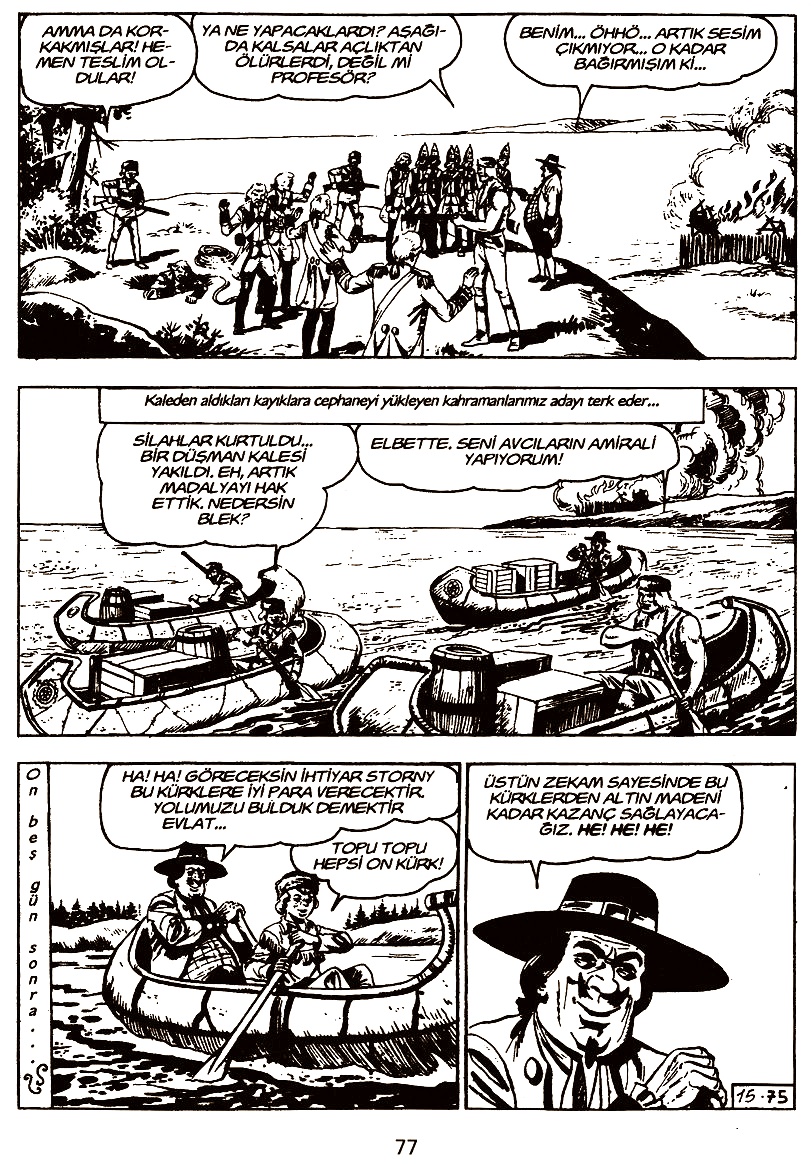The image is a detailed, black-and-white cartoon illustration, likely extracted from a magazine as suggested by the page number 77 at the bottom center. This comic-style sketch is divided into four panels: three larger ones and two smaller ones at the bottom, split in half. The scene portrays a mix of colonial and Native American figures, along with a burning fort surrounded by smoke in the background.

The top panel features a chaotic scenario of Native Americans and Redcoat soldiers amidst the burning fort. Some soldiers hold guns while others raise their hands in surrender. On the right-hand side, a large wooden fence or fort is ablaze, with smoke billowing out.

The central panel continues with the fiery fort in the background, showing people in canoes filled with barrels, boxes, and crates. The characters, depicted in active conversation, speak in a language different from English, featuring text bubbles containing words like "Amadakor," "Kamaslari," "Heman," and others.

In the bottom-left panel, a portly man with a pilgrim hat and a bemused expression sits in a canoe beside a smaller man wearing a coonskin cap. The bottom-right panel offers a close-up of the man with the pilgrim hat, who sports a pointed mustache and goatee, enhancing his somewhat sinister appearance. He seems to be speaking, though the language remains indiscernible.

Overall, this cartoon captures a historical scene with intricate details and a clear emphasis on the tumultuous interaction between colonial and Native American figures amidst a dramatic backdrop.